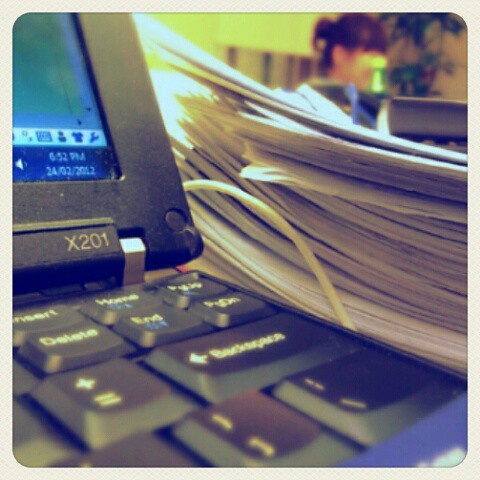The close-up image showcases the top right corner of a black X201 laptop, highlighting the backspace, plus/equal, insert, delete, home, page up, end, and page down keys. The screen displays the time as 6:52 PM and the date as February 24, 2012. Just beyond the laptop, there's a thick stack of papers, estimated to be several hundred pages. The background features a slightly blurred room with yellow walls, where a lady with a small ponytail can be seen. A small green tree adds a touch of decoration to the scene. Additionally, a cord extends from the laptop, though its destination is not visible.